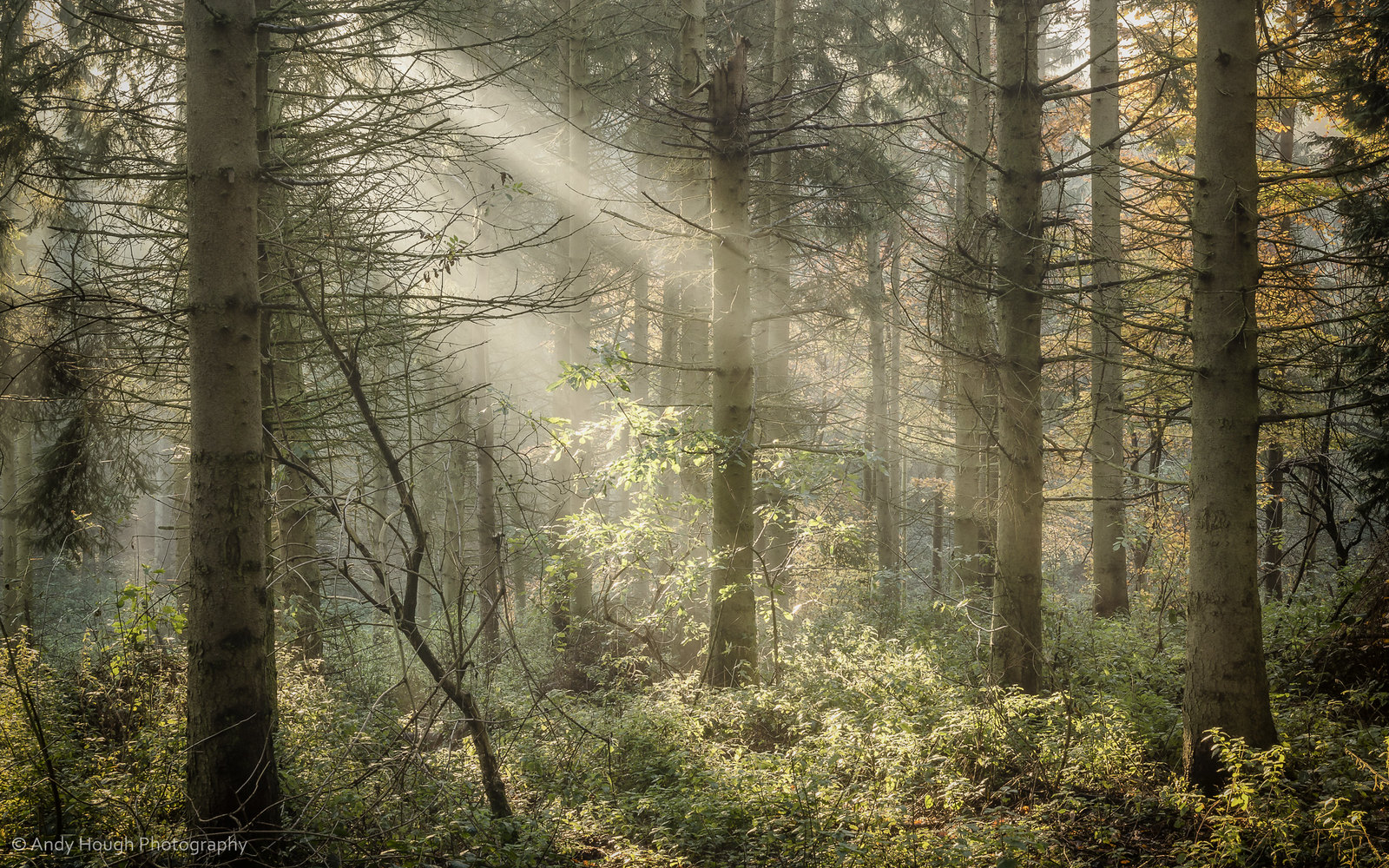This captivating photograph captures the serene beauty of a sunlit forest. The scene is filled with a multitude of trees, their long branches reaching out in various directions. The light gray bark of these trees contrasts beautifully with the lush green grass and foliage that cover the forest floor, interspersed with fallen leaves. The sunlight is shining down from the upper left, casting a dappled light throughout the forest and creating a serene atmosphere. In the background to the right, one of the trees stands out with its vibrant yellow foliage. The sunlight filters through the forest canopy, casting a soft, white-tinged gray light at a 45-degree angle from the upper left, adding depth and tranquility to the scene. In the bottom left corner of the image, the text "Andy Houch Photography" is elegantly displayed in translucent white, attributing the artwork to its creator. The overall composition emanates a peaceful, almost ethereal quality, inviting viewers to immerse themselves in the natural beauty of the forest.